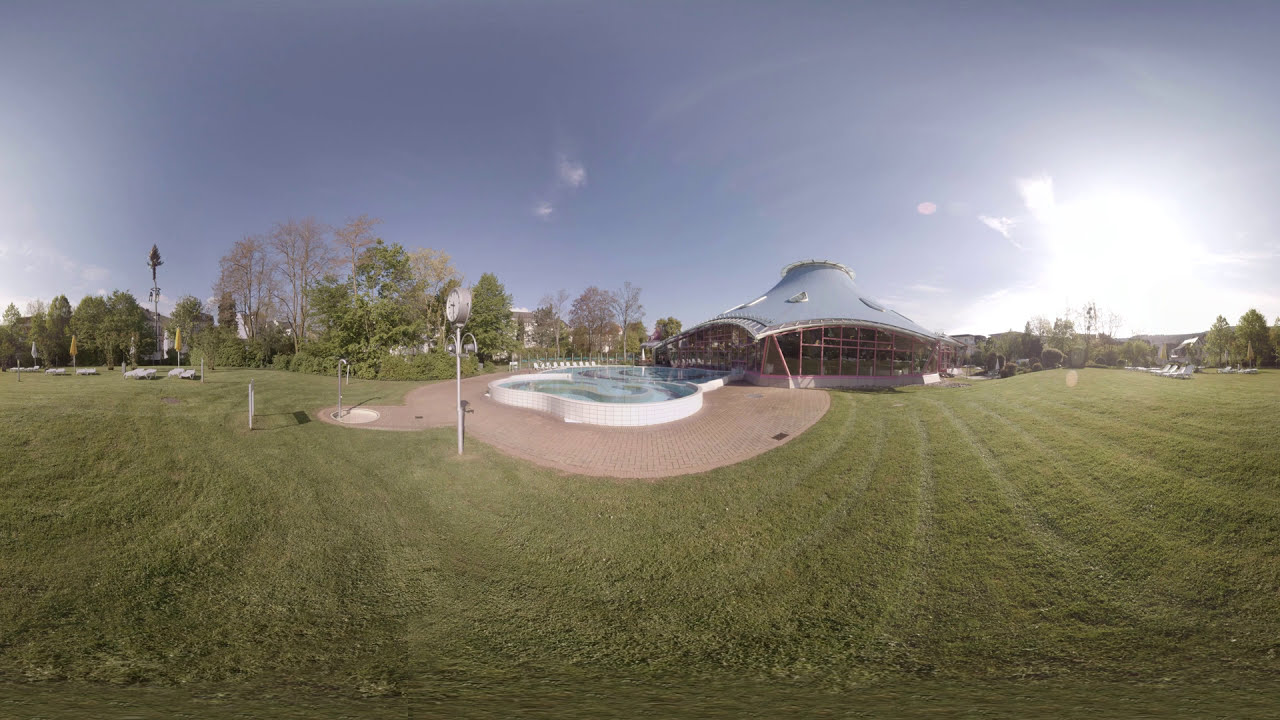This image captures a large, outdoor property under a clear, cobalt blue sky with only a couple of clouds. The vibrant grass is neatly cut with visible lawnmower tracks, creating a meticulously maintained look. At the center, a white-raised swimming pool with blue water is surrounded by a brick-tiled pavement. Nearby, a pole with a clock and an outdoor shower are visible. Just beyond, a distinctive building featuring a mix of large glass windows, a silver irregularly-shaped roof, and red support structures gives the area a unique aesthetic, reminiscent of Asian architecture. Scattered around the property, there are yellow and white umbrella-shaded tables and numerous patio chairs. The backdrop is framed by a variety of trees, adding to the serene atmosphere. The sun, positioned on the right side, adds a blinding brightness to this picturesque scene.